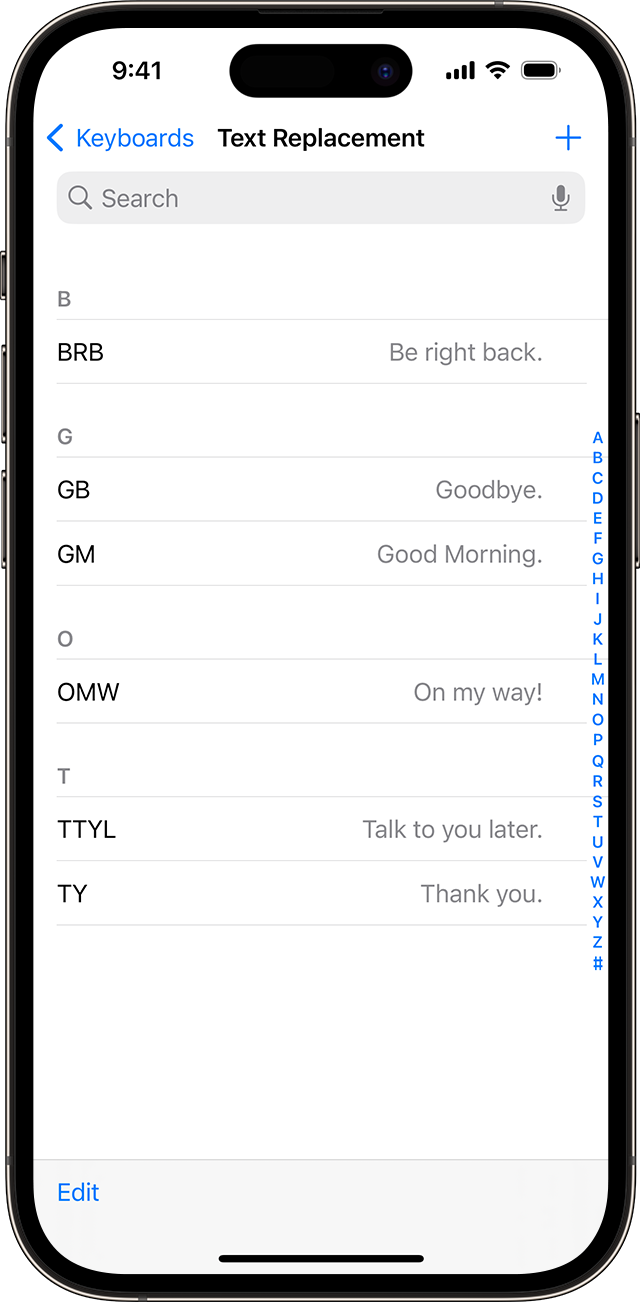This image appears to be a digitally rendered screenshot of a smartphone display, designed to showcase the appearance and functionality of an app on a virtual mobile device. The outline of the smartphone is distinctly visible, suggesting it is a product page illustration aimed at providing a visual representation of the app for prospective users.

At the top of the screen, the time is displayed as 9:41 AM on the left side, and the battery icon on the right indicates that the battery is fully charged. Centrally placed at the top is the title "Text Replacement," with a search bar situated directly below it, suggesting this is a functionality within the app.

The screen is organized similarly to a contacts list interface on a smartphone, featuring a vertical alphabet index from A to Z along the right side for quick navigation. However, instead of contact names, the list contains common text messaging abbreviations and their respective full forms.

Under the letter "B," the abbreviation "BRB" is expanded to "Be Right Back." The "G" section shows "GB" as "Goodbye" and "GM" as "Good Morning." Moving to "O," "OMW" stands for "On My Way." In the "T" section, "TTYL" is translated to "Talk To You Later," and finally, "TY" is listed as "Thank You." 

This detailed list serves as an informative guide that provides clear definitions of various common abbreviations used in text messaging, helping users understand and utilize shorthand communications efficiently.